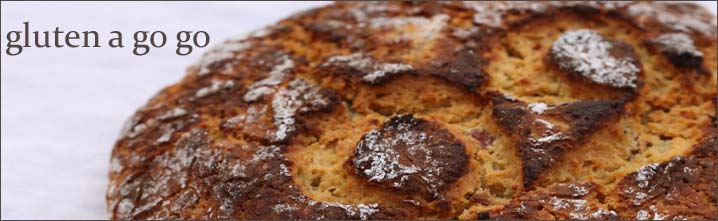The image is a wide rectangular photograph, approximately five times wider than it is tall, framed with a black outline. It depicts a close-up of a loaf of French-style bread, showcasing its circular shape and crunchy crust. The loaf is predominantly brown with a lighter shade of brown in areas where the crust did not rise as much. Notably, the top of the bread features indentations resembling a pattern of a number six or eight, creating a faint visual of two eyes and a nose. The surface of the bread is dusted with flour, more heavily concentrated on the left side and back right corner.

On the left side of the image, covering roughly 25% of the width, there is a light grey-white background, likely a table. In the upper left corner of the photograph, the text "GLUTEN-A-GO-GO" is prominently displayed in black, lowercase letters, suggesting that the bread is gluten-free.